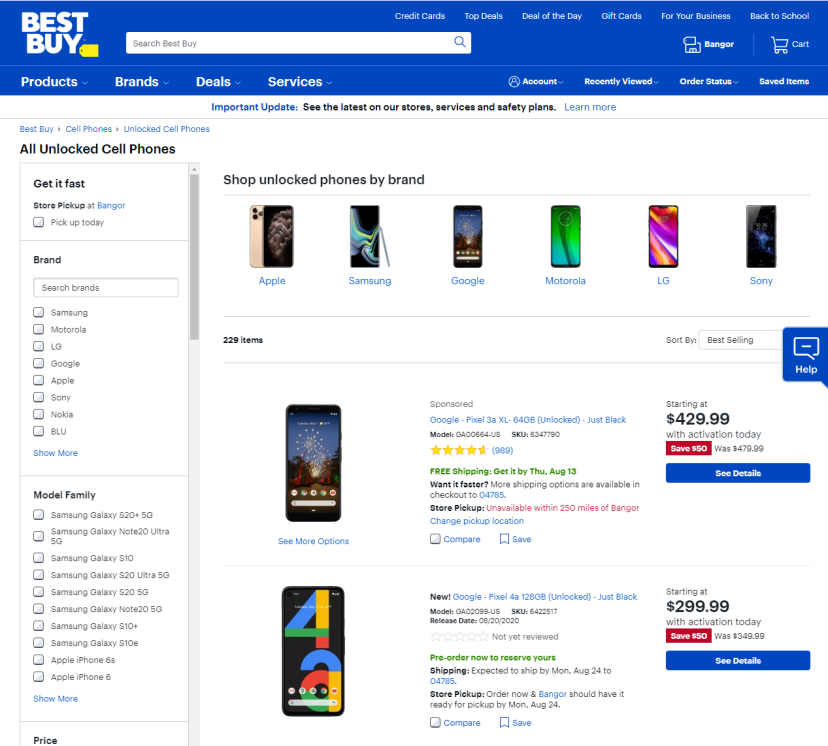On the Best Buy website, the upper left corner of the top bar prominently features the "Best Buy" logo against a blue background. The top bar also includes several horizontal menus. To the upper right, a justified menu lists options such as "Credit Cards," "Top Deals," "Deal of the Day," "Gift Cards for Your Business," and "Back to School," starting from the center and spreading outward. Below this, right next to the "Best Buy" logo on the left, is a search bar for users to search Best Buy's offerings.

Immediately beneath this search bar is another horizontal menu, which broadens the navigation options with categories including "Products," "Brands," "Deals," and "Services." On the left side of the webpage, there is a vertical menu divided into three sections, though the bottom of the price section is cut off from the view.

The main content of the page focuses on cell phones, showcasing two specific items. One of these cell phones is priced at $429.99.